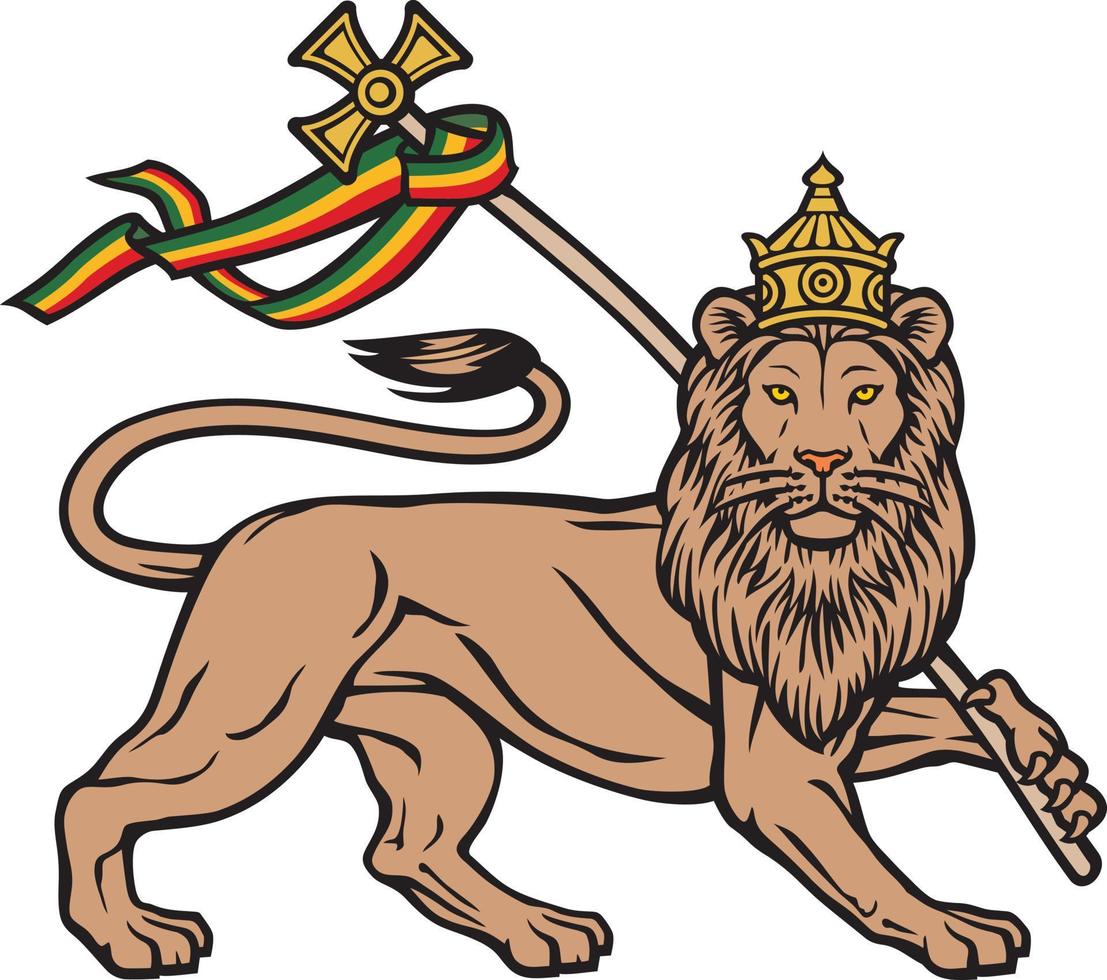In this computer-generated, animated image, a brown lion is depicted walking towards the right, but its head is turned to face the viewer. The lion has yellow eyes, a pink nose, and a black tail. Atop its head rests a gold crown with a dome and a triangular point. This regal lion holds a brown staff over its shoulder with a golden three-point cross at the top. A ribbon of red, yellow, and green is wrapped around the staff, billowing out beneath the cross as if caught in the wind. The background is solid white, placing all the focus on the detailed and majestic lion.